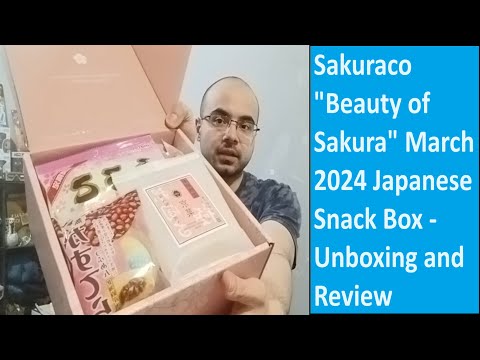The image is a screenshot from a YouTube unboxing video featuring a bald, glasses-wearing man with a nerdy appearance, dressed in a blue and gray t-shirt. He's holding up a bright pink box filled with various Japanese snacks, with some packaging displaying Japanese writing and small seed-like details. The video title, displayed in white text on a blue background on the right side of the image, reads: "Sakurako Beauty of Sakura March 2024 Japanese Snack Box Unboxing and Review." The screenshot also has black bars at the top and bottom, with shelving and a white wall in the background.